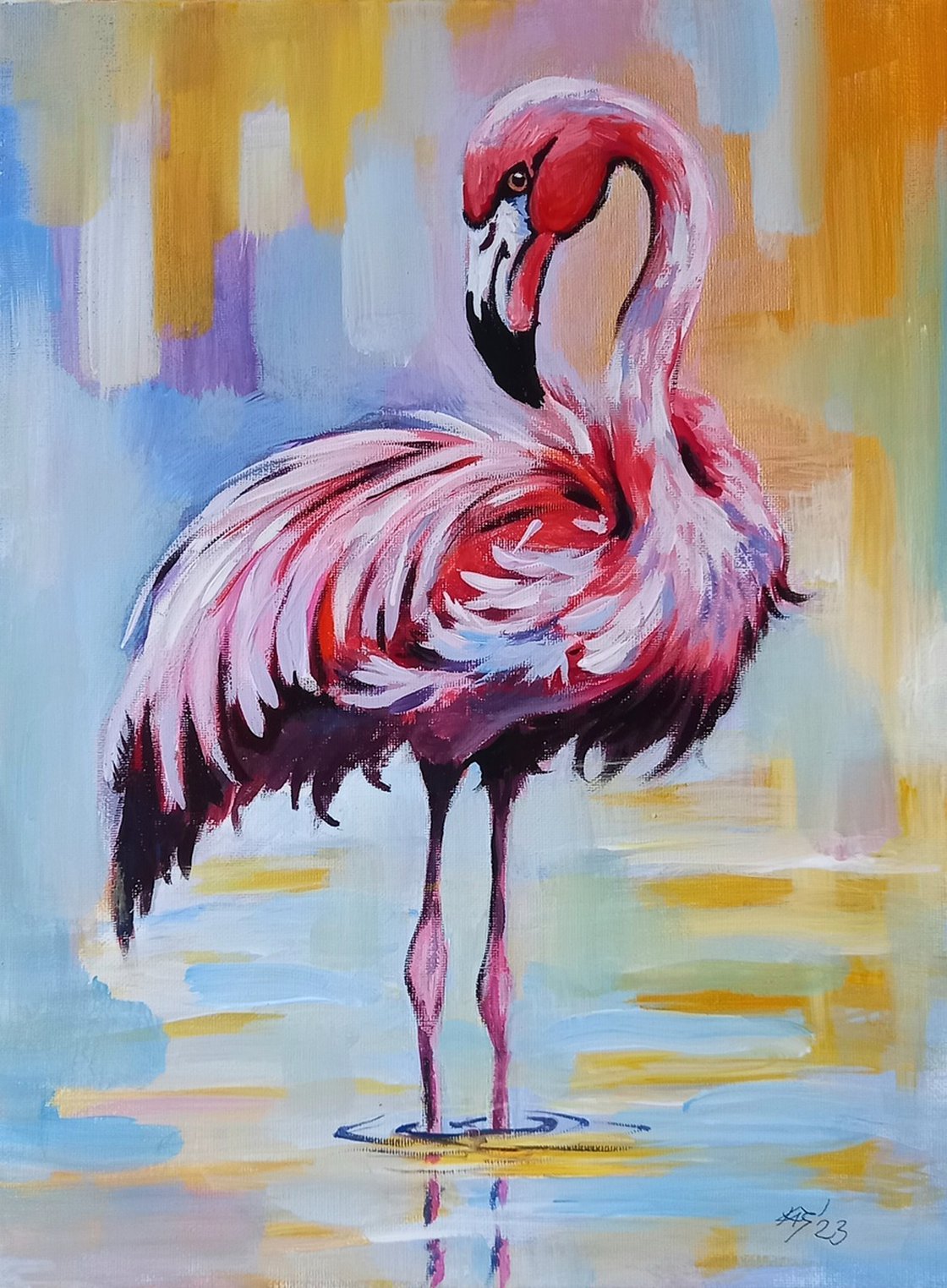The painting showcases a vibrant flamingo standing gracefully in teal water with golden reflections. The flamingo, predominantly pink, displays a mesmerizing array of colors—dark reds, whites, and subtle touches of black, notably on its large beak which also has white and pink accents. Its legs, a mix of pink and purple, create ripples in the water. The bird's neck is elegantly turned towards its back, and its striking eye, tinged with yellow and orange, gazes directly at the viewer. The background bursts with a rich palette of pastel colors—blues, yellows, purples, pinks, and even hints of green—that seem to blend and swirl, perhaps mimicking an abstract rendition of trees or buildings reflected in the water. In the bottom right corner, there is a symbol, possibly the artist’s signature, alongside the number 23. This overall scene is a feast of bright and vivid colors, emphasizing the detailed and textured appearance of the flamingo's feathers and the water around it.